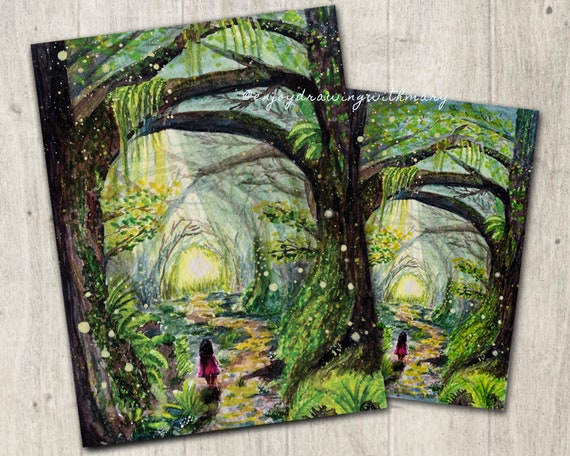This artwork features two identical prints displayed together — one vertical and one horizontal, with the vertical print placed over the horizontal, showing the full scene while the horizontal print reveals only a partial view. The scene depicts a tranquil, fantasy-inspired landscape framed by two towering trees on either side, their branches arcing overhead to create a canopied pathway. Long strips of green moss hang from these branches, enhancing the enchanted atmosphere. At the end of this passage, a radiant, bright yellow sun or light beckons, suggesting an exit to a brighter realm.

The path, a meandering dirt trail, zigzags through the scene, leading towards the sunlit background. Along this path, a small child, seen from behind, is depicted wearing a pink dress and sporting long, dark hair that falls to her waist. The child appears to be journeying into the depths of this whimsical world.

The image also contains minimal text, notably an Instagram handle "Enjoy drawing with Mary" in small, white cursive. The background wood paneling, visible in some parts, appears in a silent gray and white tone under a set of six panels, adding to the rustic charm of the presentation. The overall color palette is a harmonious blend of green, brown, black, yellow, pink, and white, enhancing the sense of a magical, yet serene, woodland path.